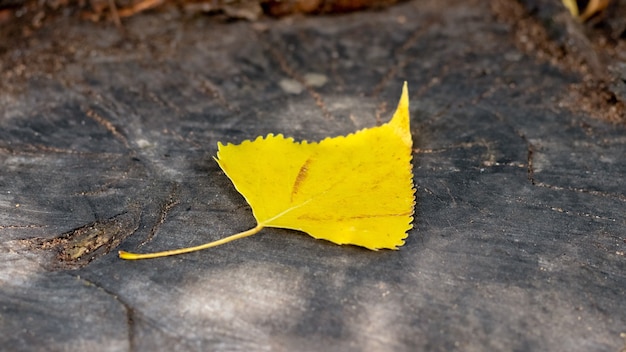This detailed photograph, taken in landscape layout, showcases a bright yellow, triangular-shaped leaf lying on a weathered, cracked black pavement. The leaf, which appears to have aged into its vibrant yellow hue, features jagged, fringed edges and a thin yellow stem that extends toward the lower left corner of the image. The ground beneath the leaf is adorned with brown dirt, small rocks, and debris, adding texture and depth. Sunlight gently illuminates the scene, highlighting subtle orange-brown veins running diagonally from the base to the leaf's center. Although some other parts of the ground are blurry, the leaf itself is the sharp focal point, providing a striking contrast against the dark, rugged pavement.